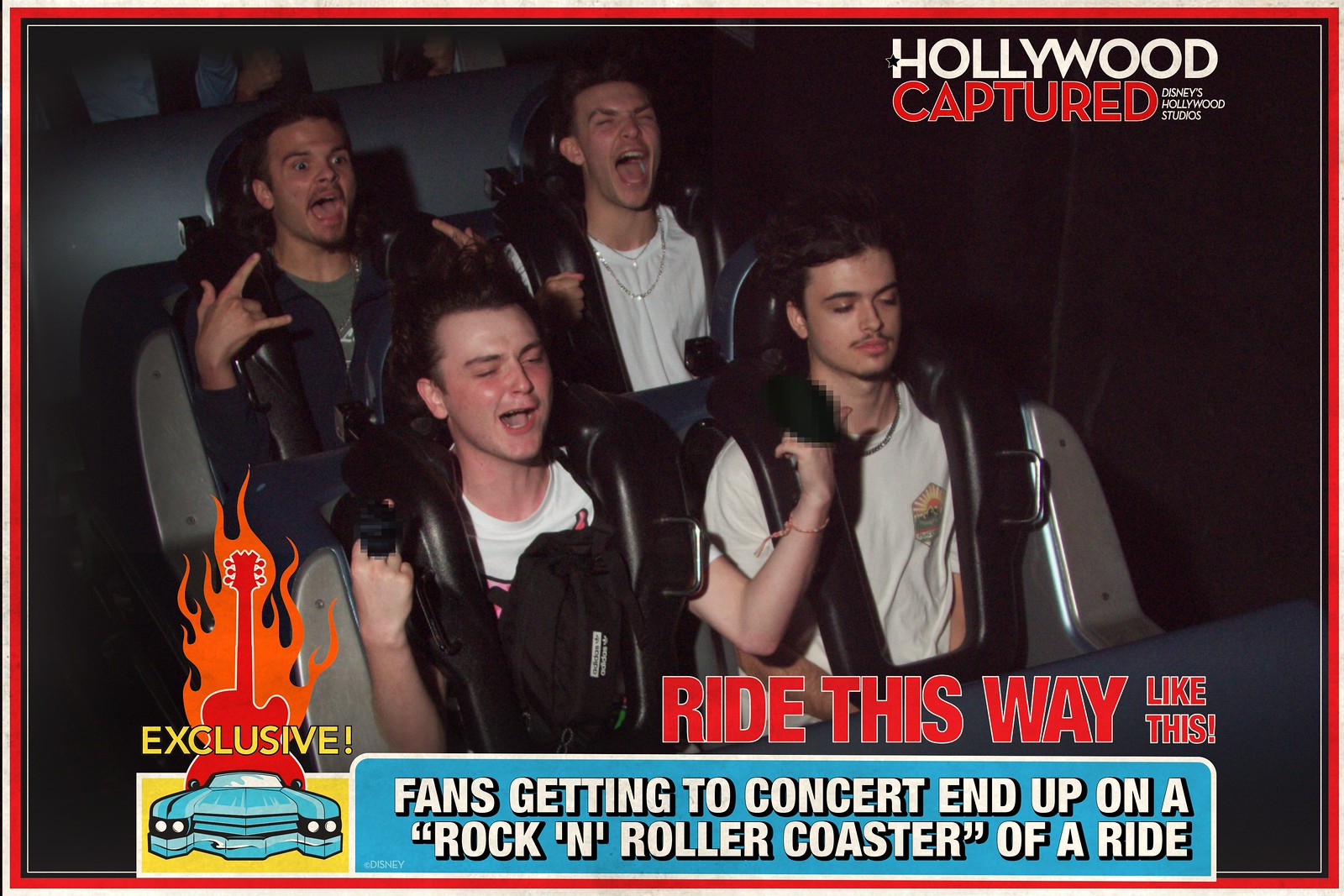The image is a promotional poster for the Aerosmith Rock 'n' Roller Coaster at Disney's Hollywood Studios. It features a background picture of four young men strapped into a roller coaster, three of whom are visibly excited with wide-open mouths and closed eyes, while one person appears calm. The top right corner of the image contains the text "Hollywood Captured" in white and red against a black background, followed by "Disney's Hollywood Studios." At the bottom left, there is a drawing of an electric guitar engulfed in orange flames, resting on top of a blue car, with the word "exclusive" written above it. To the right of this drawing, the text reads "Ride this way like this," and below these elements, in white lettering on a blue background, it states, "Fans getting to concert end up on a rock and rollercoaster of a ride." The poster is framed with a red and white border.